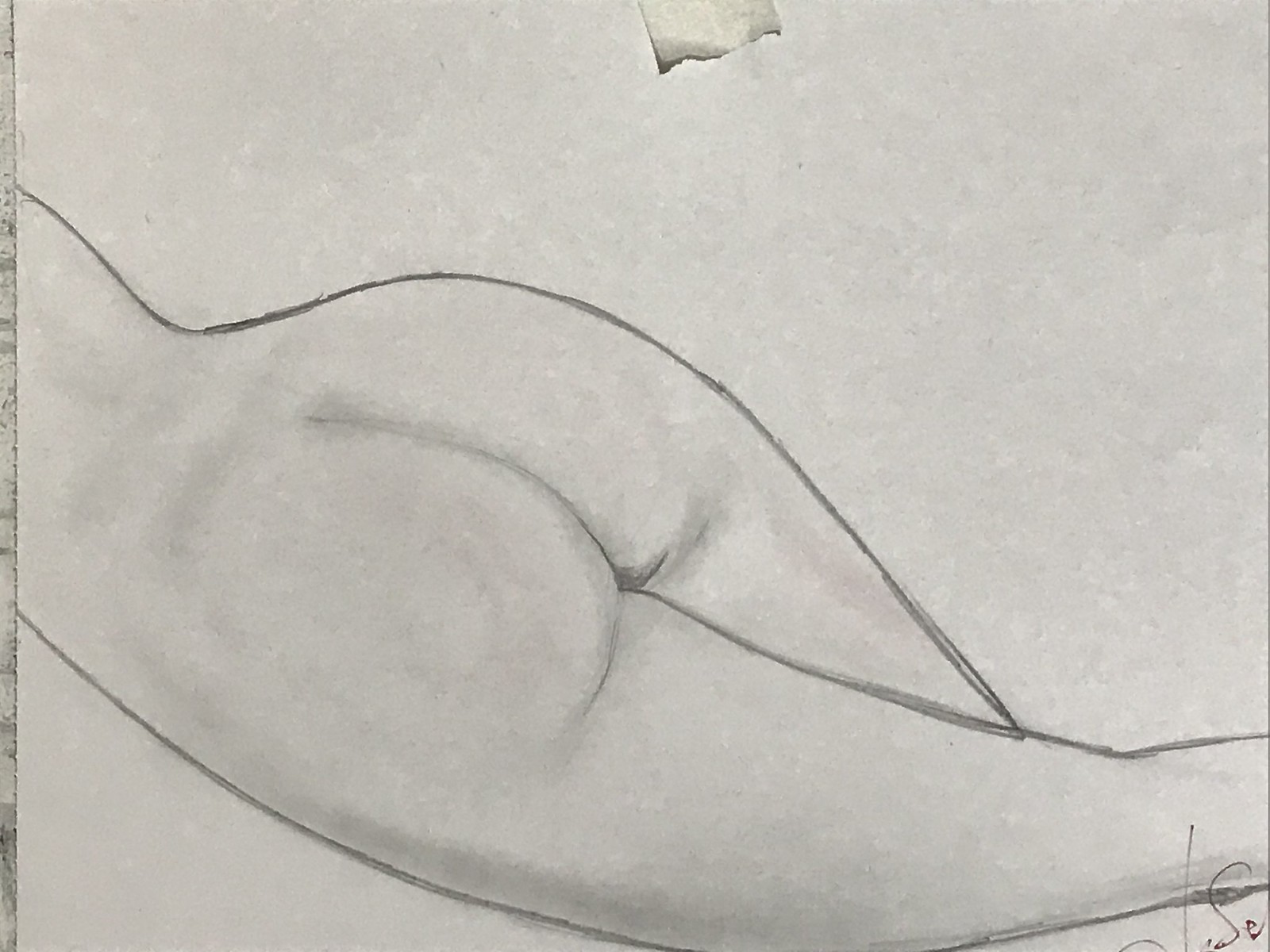This artwork is a detailed pencil or charcoal drawing, rendered on off-white paper with a tear visible at the top center and a sliver of a stone surface peeking out from the left edge. The sketch captures the lower half of a slender, nude woman's body as she lies on her stomach. The composition extends from the mid-back down to the knees, accentuating the curve of her hips and legs. Her legs are crossed, creating a dynamic twist in her posture. The sharp outlines of her form contrast with the subtler, shaded interior, emphasizing the natural creases and curves of her buttocks and thighs. The bottom right corner of the image features a partial, pencil-drawn signature, with the visible last name starting with "SO." A piece of white tape secures the drawing at the top, adding a casual, unfinished touch to this intimate, evocative depiction.